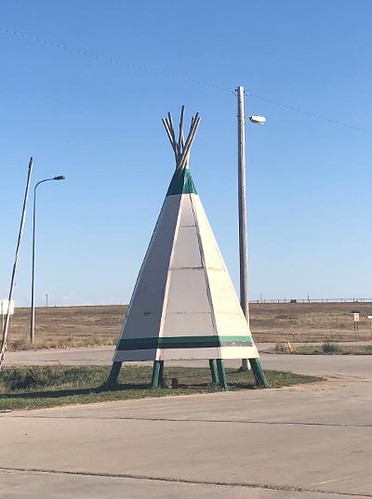This detailed outdoor photo depicts a classic, triangular-shaped Native American tipi positioned centrally on a small patch of grass or dirt, adjacent to a stone or asphalt pavement. The tipi features six wooden poles that converge at the top, where they are tightly wound together. Its exterior exhibits a unique color pattern: predominantly white, with a blue-green top, a blue-green stripe at the bottom, and a black stripe directly below it. To the right and behind the tipi, a sidewalk leads to a roadway, and in the background, multiple street signs, street lights, and power lines traverse the sky. The surrounding landscape is characterized by dry grasslands, open fields, and scattered weeds, indicative of an arid, countryside region. The scene appears to be captured midday, under a clear sky with colors including blue, light blue, white, green, brown, tan, and gray, contributing to the overall atmosphere of the image.